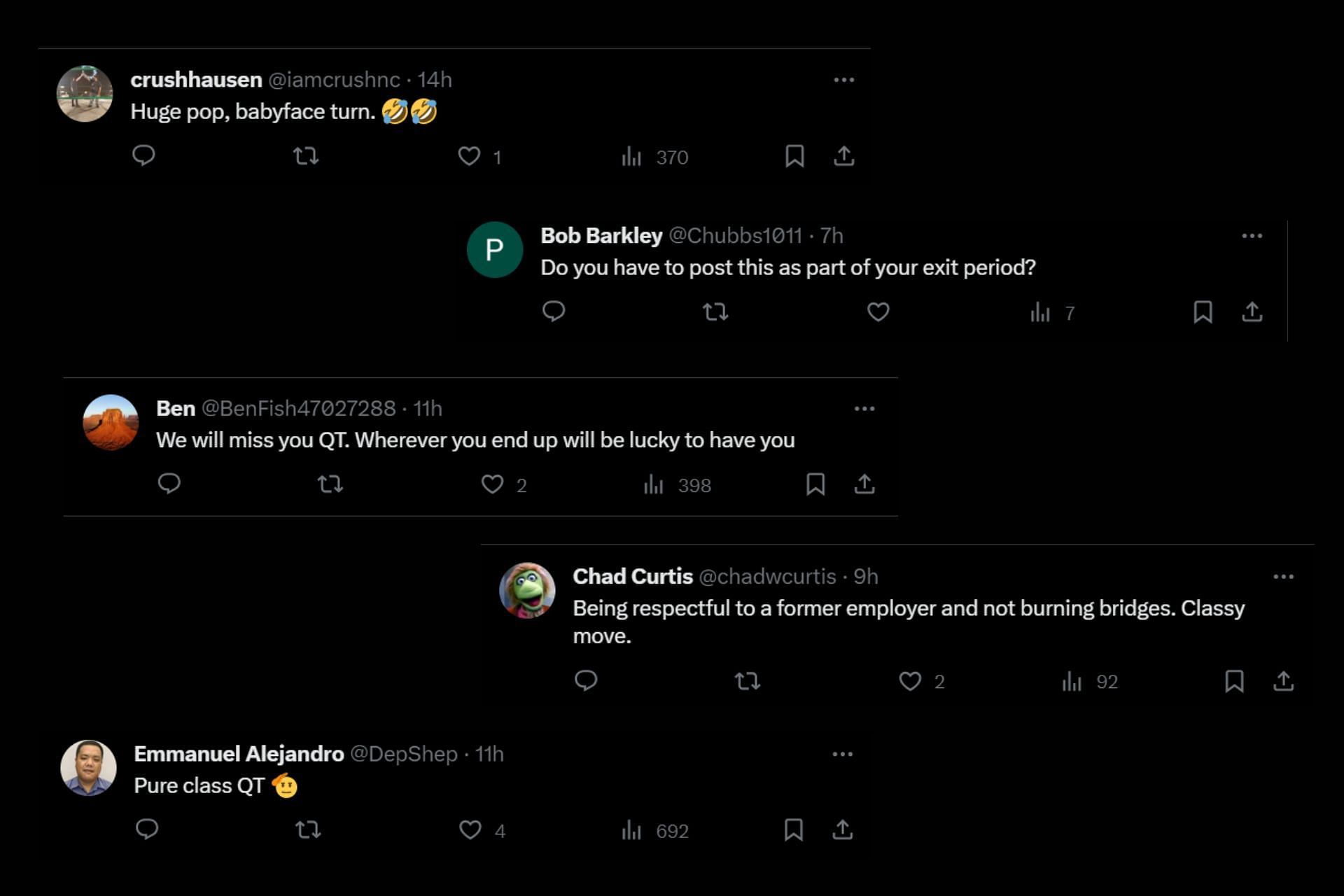The image features a series of stacked comments on a black background, organized in a left-aligned format. 

1. At the top is a comment by Crash Hosan, whose account handle is @IAmCrashNC. The text appears in white font and is accompanied by a profile picture to the left of the username. The comment, posted 14 hours ago, reads: "Huge pop, baby face turn," followed by two crying emojis.

2. The second comment is from Bob Barkley, with the handle @Chubbs101. Seven hours ago, he wrote: "Do you have to post this as part of your exit period?"

3. Below that, a comment by Ben expresses sentimentality: "We will miss you, cutie. Wherever you end up, we'll be lucky to have you."

4. Chad Curtis follows with a comment emphasizing respect: "Being respectful to a former employer and not burning bridges – classy move."

5. At the bottom, a comment by Pure Class Cutie simply adds an additional layer of admiration.

Each comment contributes to a narrative of departure, respect, and admiration.